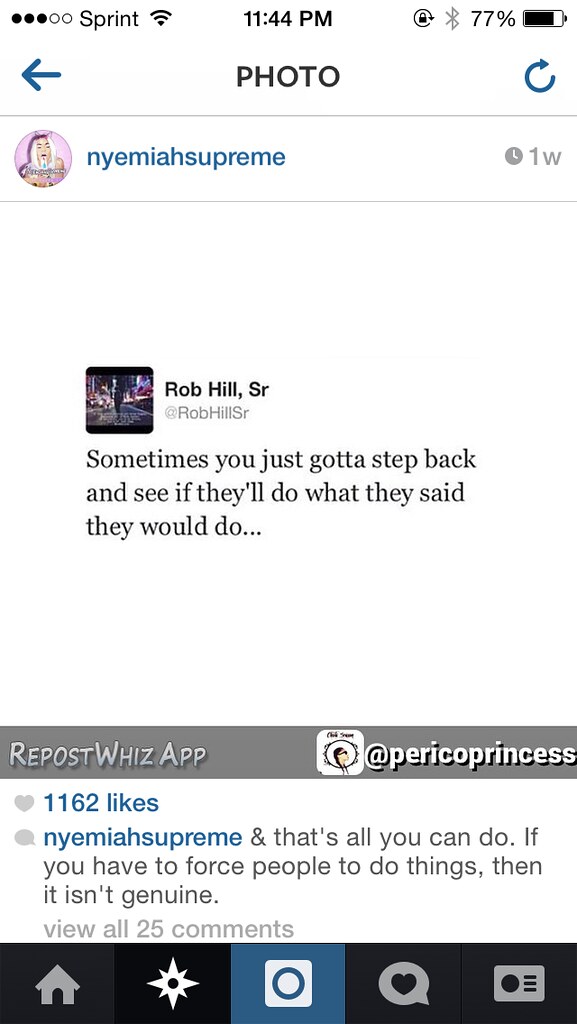The image is a screenshot from a cell phone, showing the time as 11:44 PM at the top center, with a 77% battery charge on the top right, and the carrier name, Sprint, to the left. Just below the time, it says "Photo" in black letters. On the left side below the time, there is a blue arrow pointing to the left, and a blue refresh icon to the right. The screenshot features a small circular profile picture of a woman with a purple background, labeled as Nehemiah Supreme, with an indication that this was posted one week ago (marked by a clock icon and "1w").

Centered beneath this profile information is a small rectangular image featuring text by Rob Hill Sr. which reads, “Sometimes you just got to step back and see if they'll do what they said they would do.” This post is tagged with “Rob Hill, Sr” and at the bottom of the screen, it shows the Repost Whiz app used to repost this quote. Notably, the post has garnered 1162 likes. Nehemiah Supreme commented on this post saying, "And that’s all you can do. If you have to force people to do things, it isn’t genuine." Below this interaction, there is an option to view all 25 comments on the post. At the very bottom of the image, typical phone interface symbols such as the home button are visible.